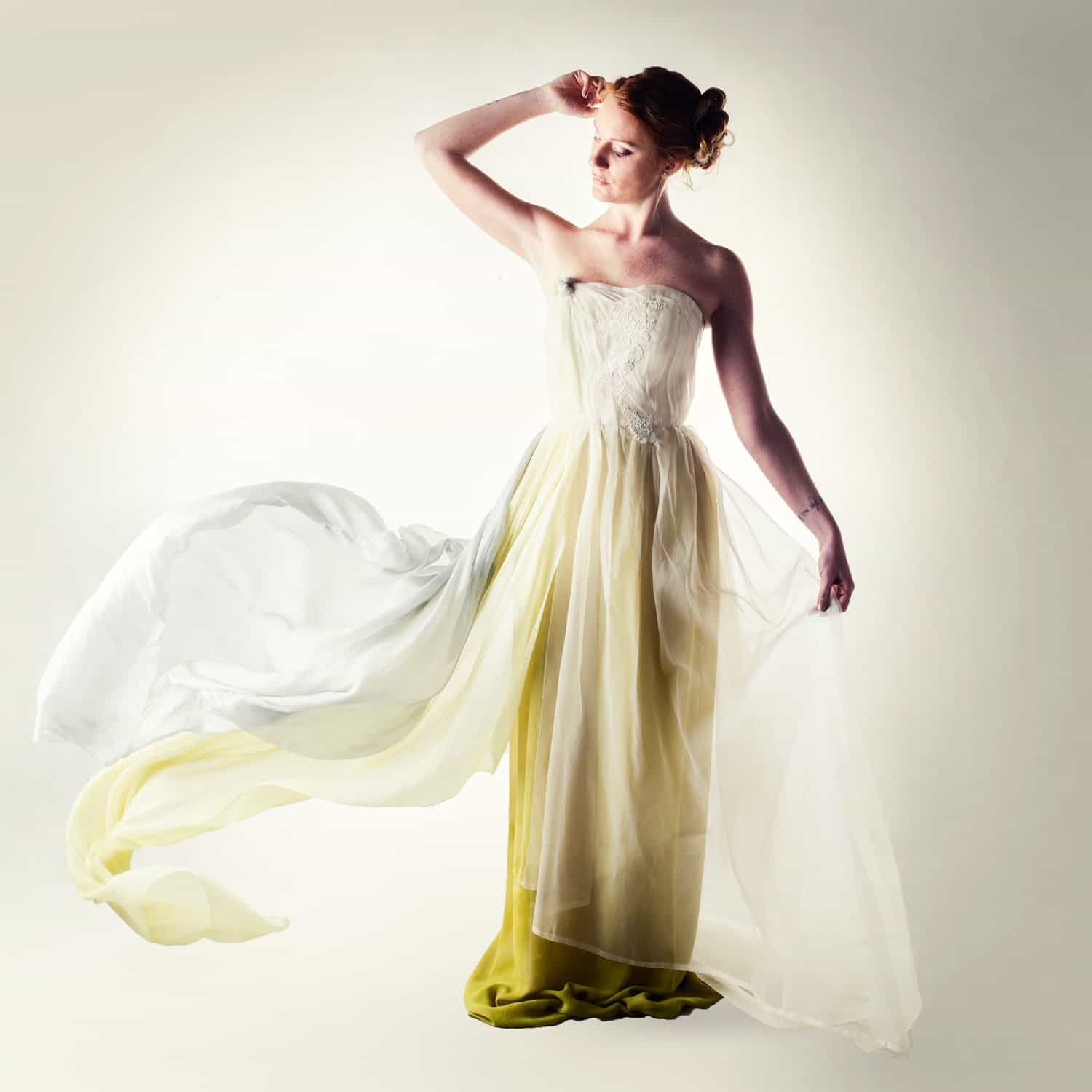In this well-lit studio photograph, a beautiful, fair-skinned woman with reddish-brown hair is modeling a strapless wedding dress that gracefully combines white and yellow. The top of the dress is knitted and white, while the bottom is a flowy, flared yellow adorned with elegant white veils. Her hair is meticulously pinned up, further highlighting her poised elegance. The model's right arm is bent at a 45-degree angle, raised and curved gracefully around her head, while her left hand gently holds one of the billowing veils, subtly lifted by a breeze from a hidden fan. She has her eyes closed, and the setup, with the studio's soft and neutral background shades, expertly accentuates the dress's appeal. This image clearly captures the essence of a high-fashion dress advertisement or possibly a serene, modern bridal photoshoot.